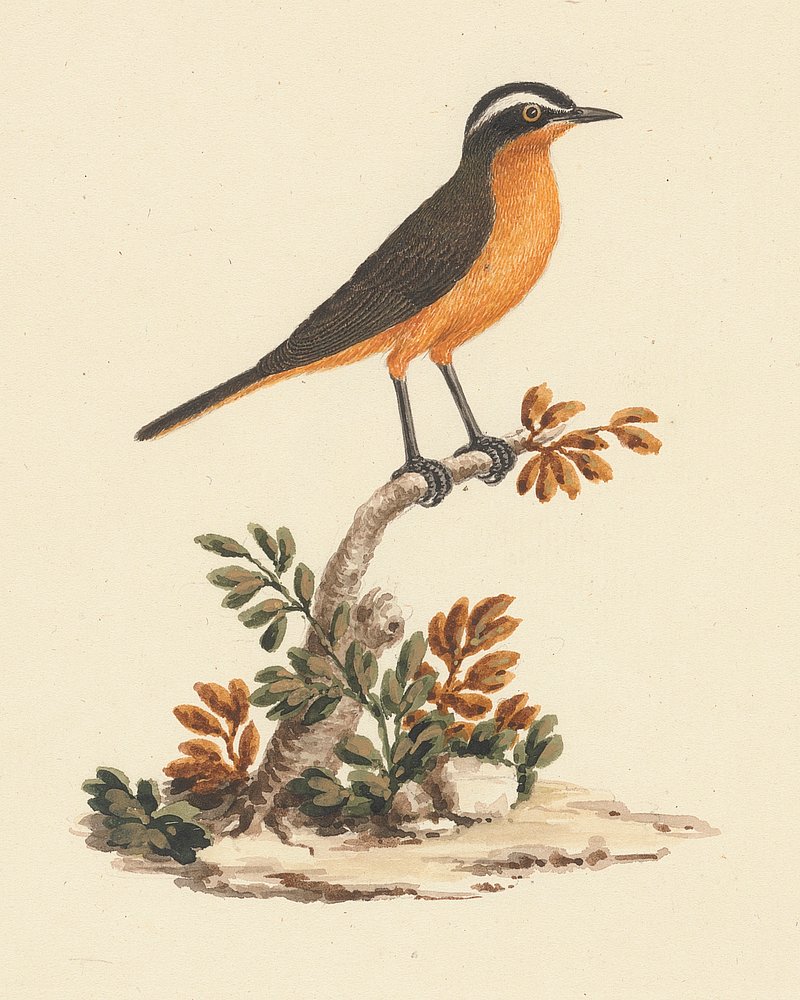The artwork features a detailed illustration of a bird perched on a light brown branch that extends from a patch of earth at the center of a light brown background. The branch curves to the right and is adorned with a mix of light brown, dark brown, and green leaves. A pile of dirt and two rocks anchor the base of the branch in the earthy patch. The bird, with its intricate coloration, has a brown tail, a predominantly orange-tinted underbelly, and brown wings with some areas of black feathering. A distinct white stripe extends from its beak over its eye to the back of its head. The bird's small black beak, legs, and claws stand out against its slightly lighter brown body. Positioned almost flat at the top of the branch, the bird is oriented to the right, showing its side profile and seemingly focused gaze in the same direction. The overall theme of the artwork suggests an autumnal setting, highlighted by the amber and green tones of the leaves. The image combines natural elements with a serene, fall-inspired palette.